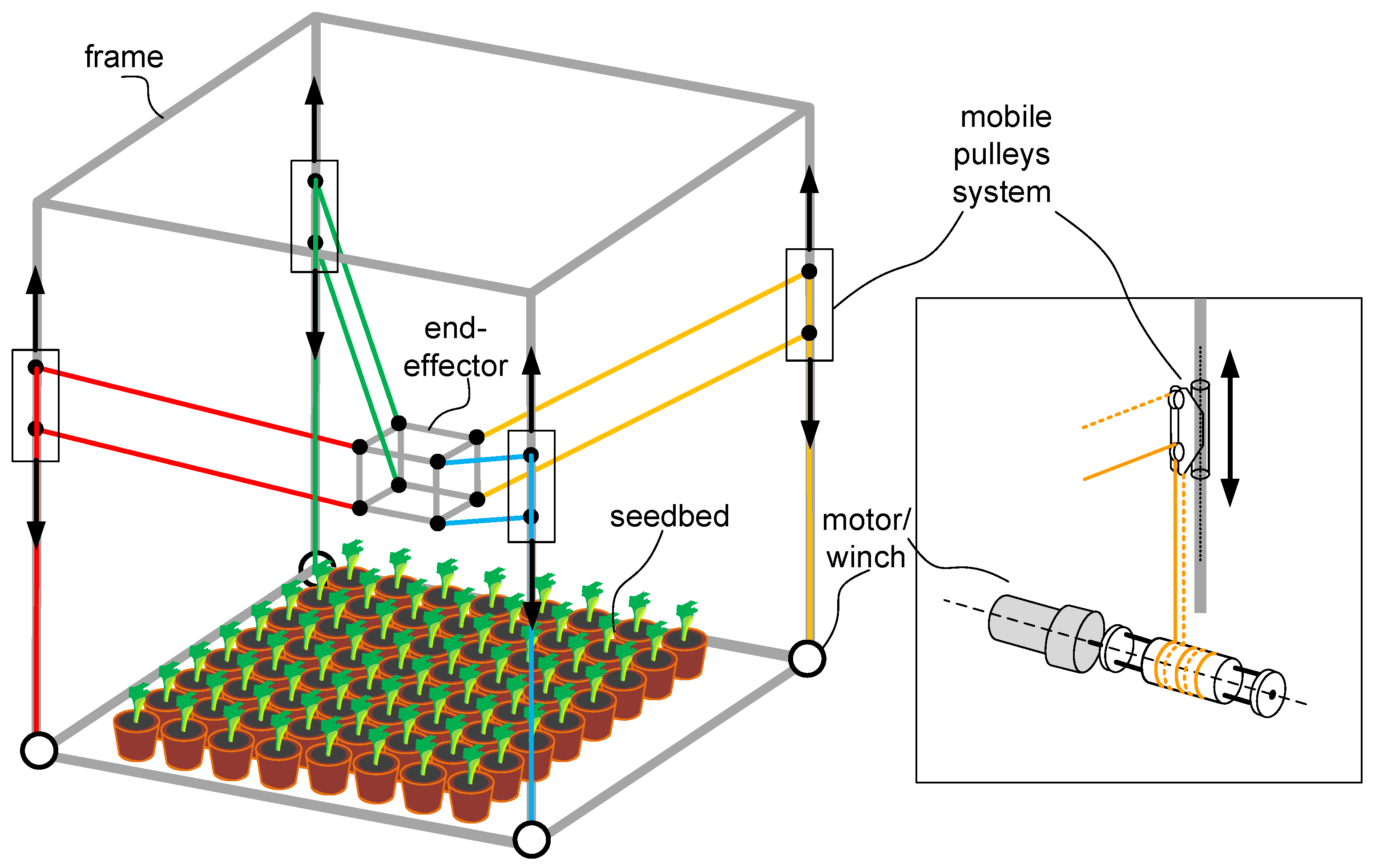This image is a detailed graphic representation of a plant management or growing system, likely set within a greenhouse or a factory environment. Central to the image is an eight-by-eight grid of small maroon pots, each containing a bit of green sprouting from the soil. The pots, totaling 64, are densely packed together within a clear 3D cube, whose sides and edges are delineated in gray.

Within this cube, parts are labeled for various components integral to the system. Suspended exactly in the middle of the cube is a smaller labeled "end-effector." Adjacent to this main graphic is another smaller diagram labeled "mobile pulleys system," which features a motor and winch. This secondary system is depicted with metal elements connected by various colored lines, including blue, red, green, yellow, and black.

The overall setup appears to be an advanced, mechanized plant-growing system with components designed to automate the cultivation process, including elements such as the frame, seed bed, and mobile pulley system. The image is set against a plain white background, emphasizing its purpose as a technical diagram without any real-world distractions.